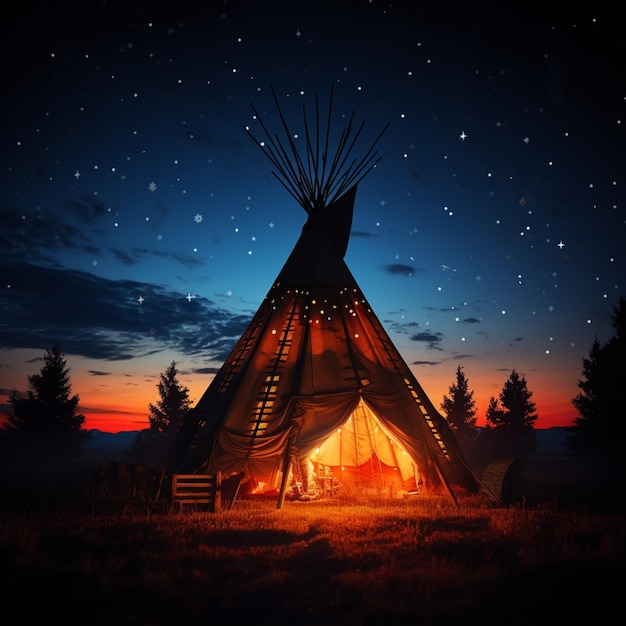This image depicts a large, traditional teepee at night set against a striking evening sky. The teepee, tan in color and topped with wooden stakes, stands prominently in the center of the scene with its fabric illuminated by a fire inside, casting a warm, yellow and reddish-orange glow. The open front of the teepee allows us to glimpse inside, where shadows dance, and suggests the presence of someone nearby. Surrounding the teepee are scattered pine trees, blending into the twilight. The sky is a mesmerizing gradient, transitioning from orange near the horizon to a deep, dark blue dotted with stars, some appearing slightly larger than usual—hinting at a digital enhancement. Clouds are faintly visible against the darkening sky, which contrasts beautifully with the grassy foreground.